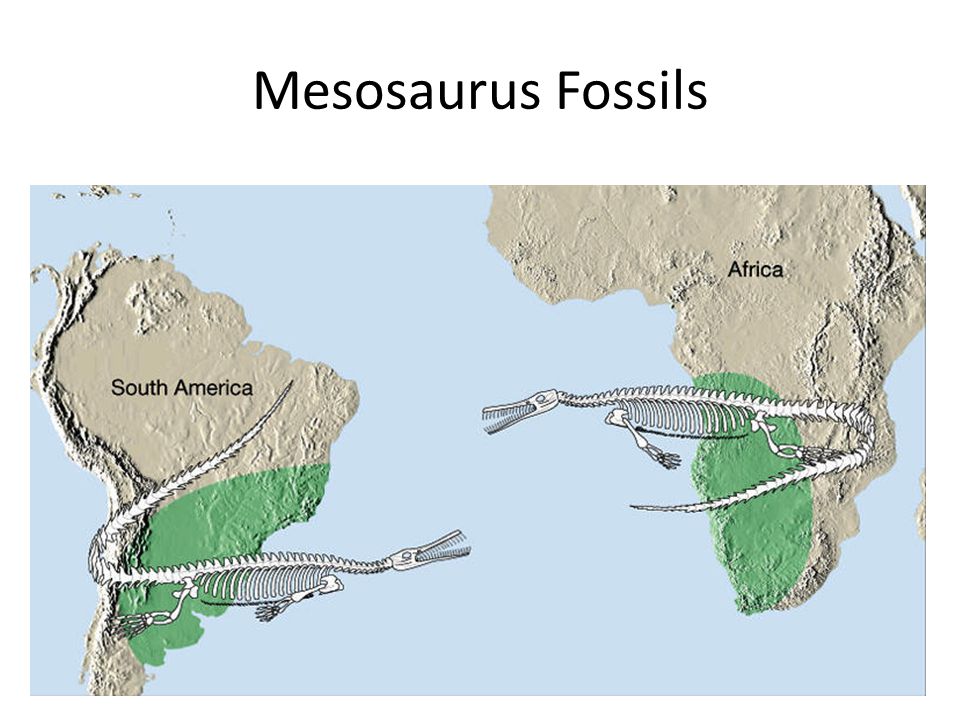This image is a detailed PowerPoint slide titled "Mesosaurus Fossils" in black sans-serif text. Below the title, there's a map featuring South America and Africa, separated by the Atlantic Ocean. Sections of the southern regions of both continents are highlighted in green, while the rest are in beige. Overlaid on these green areas are black-and-white cartoon images or diagrams of Mesosaurus skeletons, depicted as crocodile-like fossils facing each other across the ocean. This visual representation suggests that Mesosaurus fossils have been discovered in these highlighted regions, highlighting a historical connection between the two continents, possibly from the time when they were part of a single landmass. The ocean is illustrated in light blue, further emphasizing the separation of the landmasses. The map is clearly labeled, making it a concise educational tool for topics in archaeology or paleontology.